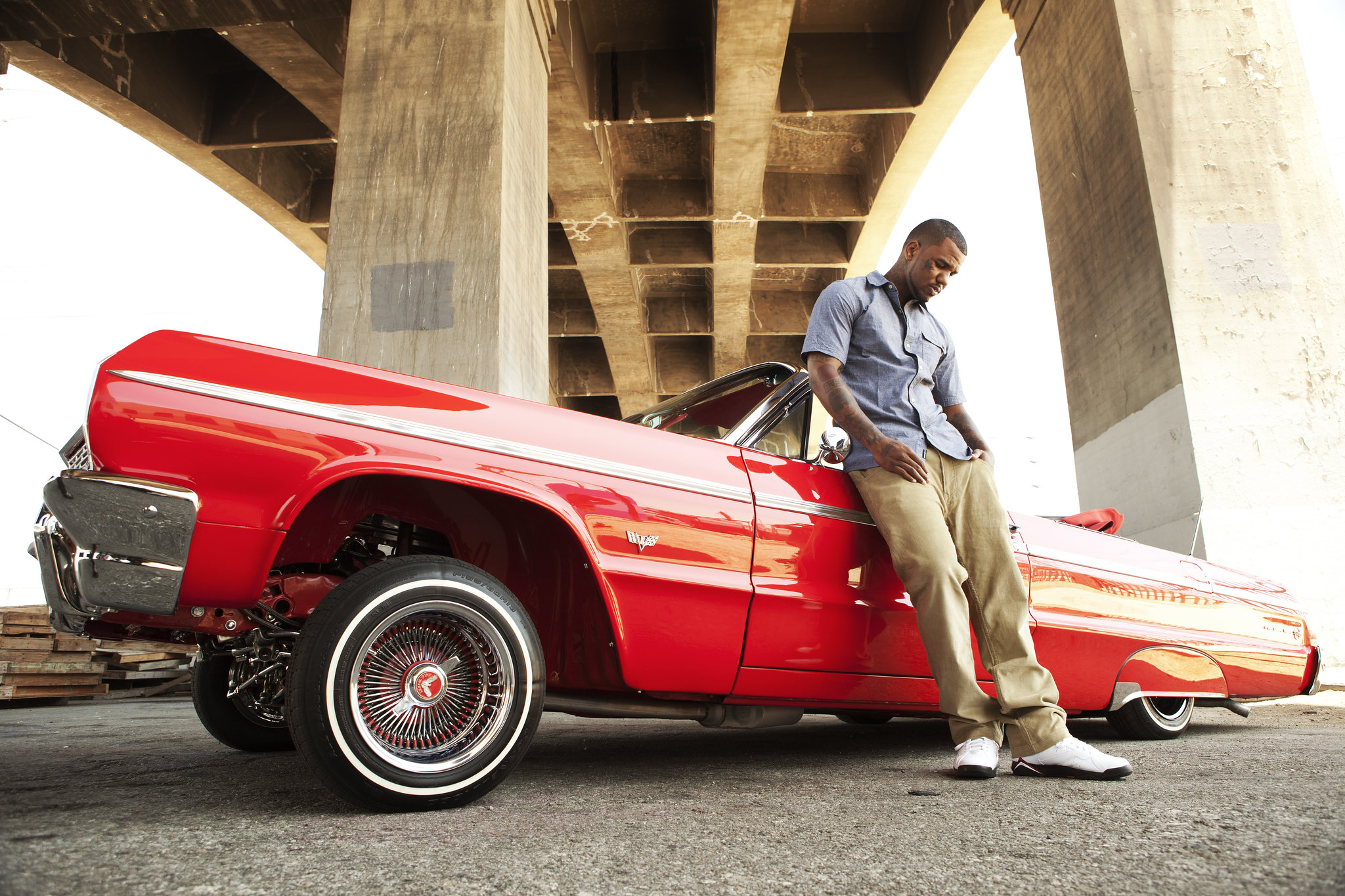A young man with a dark complexion and very short black hair, possibly African American or Hispanic, leans on the driver’s side door of a cherry red lowrider convertible under a highway overpass. The car, with its roof down, is distinguished by a silver stripe running from front to back and metallic silver hubcaps. The front of the car is elevated by a hydraulic system, giving it a tilted appearance like a boat, with the rear end sitting much lower. The man, wearing a short-sleeve button-up shirt in dark blue or bluish-gray, khaki pants, and white shoes, stands with one hand in his pocket while looking down. His hands and possibly his face are adorned with tattoos. The setting includes the light gray asphalt below, marked by rocks and oil stains, and a bridge overhead supported by large concrete pillars with multiple recesses. To the left, construction leftovers like large wooden planks or concrete slabs are visible. Sunlight filters through, casting light into the scene.